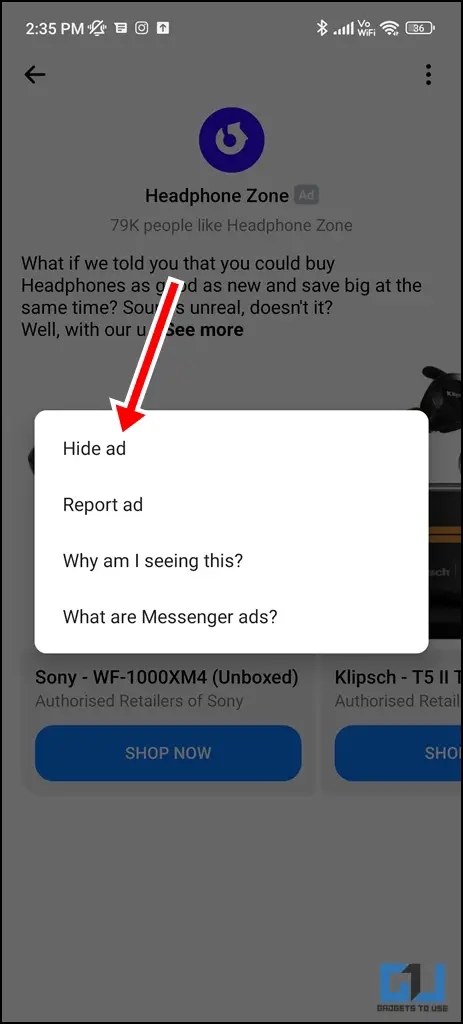In a vertically rectangular screenshot taken from a cellphone, a white pop-up window occupies the center, causing the active page in the background to appear grayed out. In the upper-left corner, the "Headphone Zone" text is visible, alongside the time reading 2:35 p.m. The status bar displays multiple icons: an alarm tone off icon, a text message icon, the Instagram icon, and an upward arrow icon. In the upper-right corner, icons for Bluetooth, cell signal strength, Voice over WiFi (VoWiFi), WiFi connectivity, and battery level are visible.

The pop-up window in the center contains four lines of text options: "Hide Ad," "Report Ad," "Why am I seeing this?" and "What are Messenger Ads?" A prominent red arrow is placed over the image, extending from just above the pop-up window and pointing directly at the "Hide Ad" option.